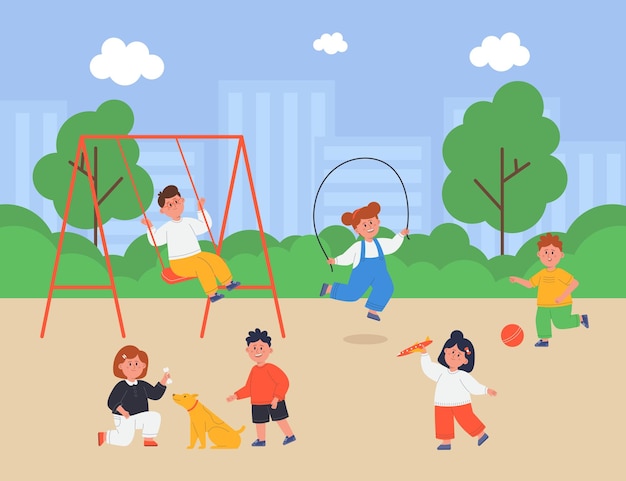The image is a vivid digital graphic of a lively playground scene under a blue sky dotted with white clouds. A cluster of buildings with a mix of blue and white colors forms the backdrop, interspersed with a few trees and bushes. The playground itself is bustling with activity: a swing set painted red sits towards the left, with a child wearing a white shirt and yellow pants joyously swinging. Nearby, a girl in a blue jumpsuit with bib overalls and a white shirt is energetically jumping rope. Another child kicks a ball to her right. On the bottom left, two kids and a tan dog with a red collar engage in a cheerful interaction. One child, kneeling in a black shirt, white pants, and orange shoes, appears to be offering something to the dog. Beside them, another child in an orange sweatshirt, black shorts, and blue shoes seems ready to pet the dog. To the bottom right, a child in a white shirt and orange pants is enthusiastically playing with a toy airplane. Overall, the scene is a vibrant depiction of children enjoying a day at the park, framed by the playful mix of green, white, orange, dark yellow, black, beige, and dark green colors.